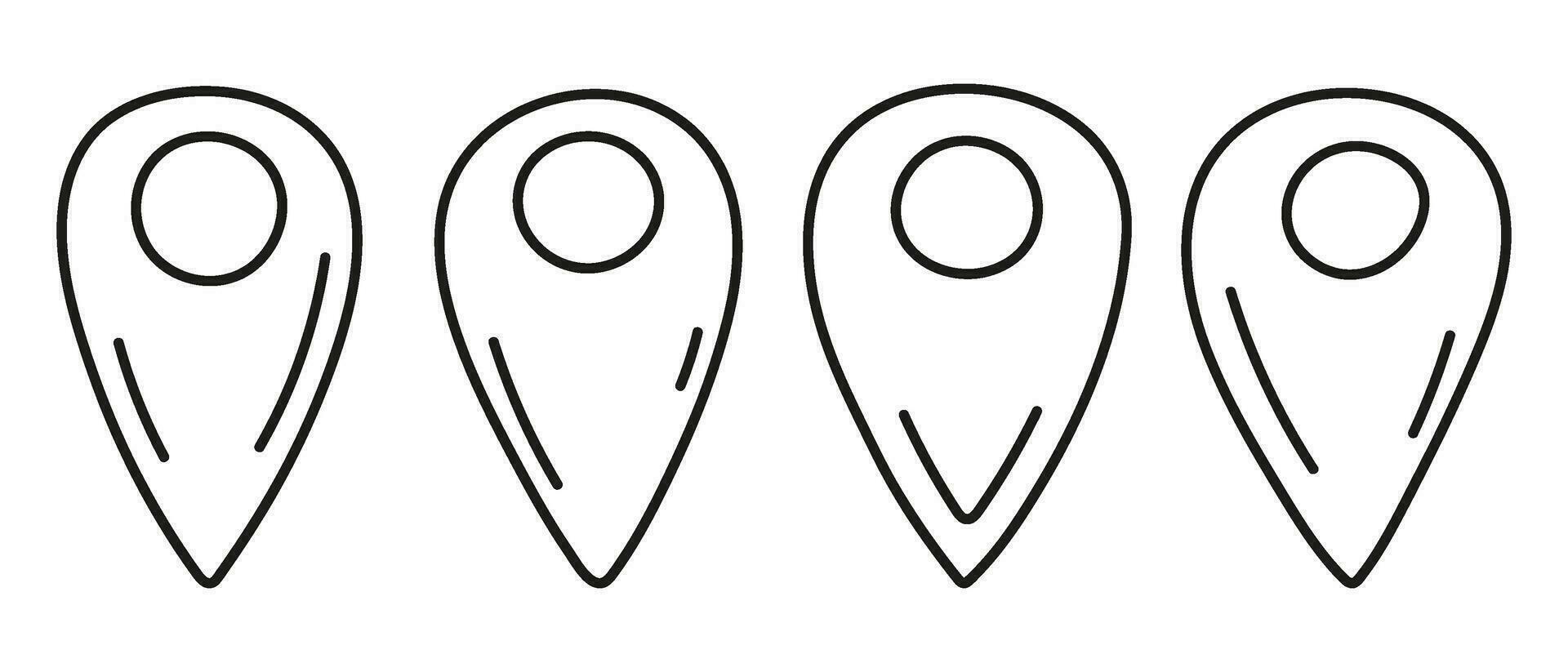The image depicts a graphic drawing of four planchettes, resembling guitar picks, all set against a white background. Each planchette adopts an upside-down teardrop shape, with the bulbous end oriented upwards and a circle situated near the top. Despite their similar overall design, the planchettes differ based on the interior lines. The first planchette features a shorter line on the left and a longer line on the right. The second planchette shows a longer line on the left and a shorter line on the right. The third planchette is marked by a triangular shape with its base missing at the pointed end. Finally, the fourth planchette has a long line on the left side and a shorter line on the right side. The overall illustration is created using black marker lines on a stark white background, with the planchettes' interiors remaining white except for the distinct interior lines and borders.